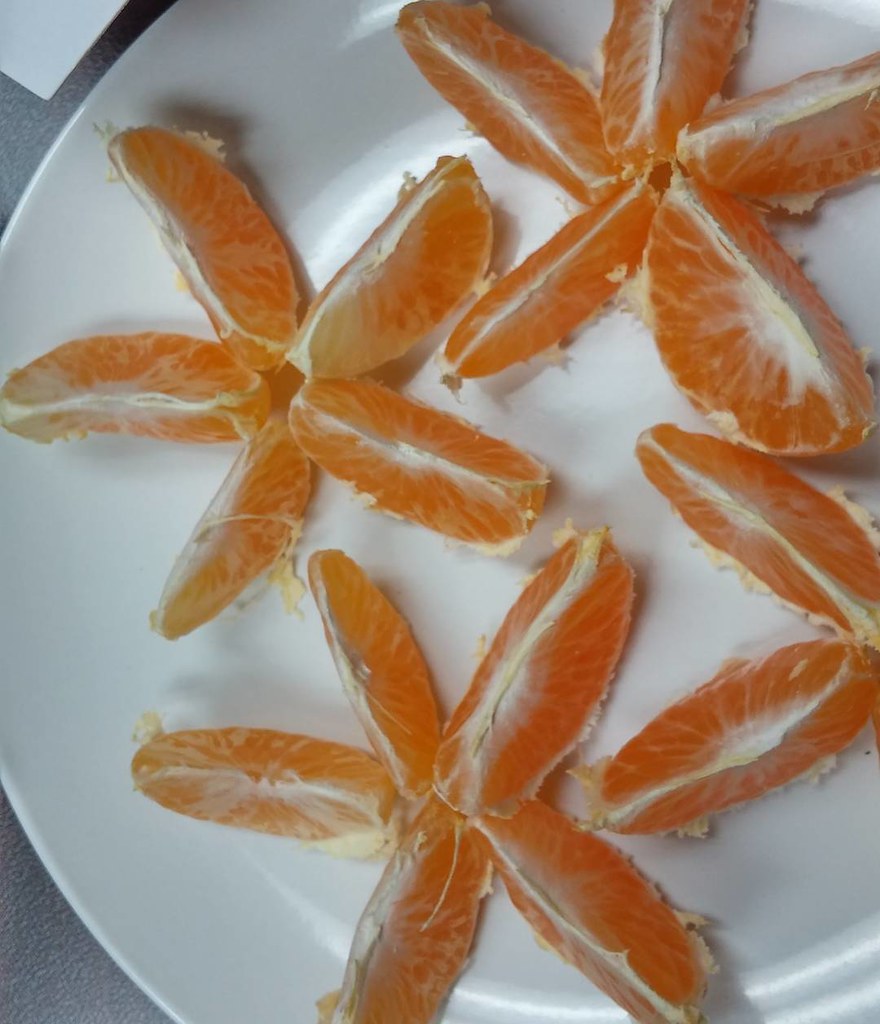This close-up image features a white ceramic plate with slightly raised edges, placed on a rough, gray countertop. The main focus is on the peeled orange slices arranged meticulously in a star formation. Each star consists of five slices, positioned at roughly the 12, 2, 4, 7, and 10 o'clock positions. In the image, there are four such star-shaped arrangements, though the bottom right formation is partially obscured, showing only two slices. The vibrant orange flesh of the citrus slices contrasts sharply against the white plate, with some pieces showing delicate membrane strands. Faint shadows are cast by the orange slices, adding depth to the composition. A hint of a white wall can be seen in the upper right corner, further framing the scene.